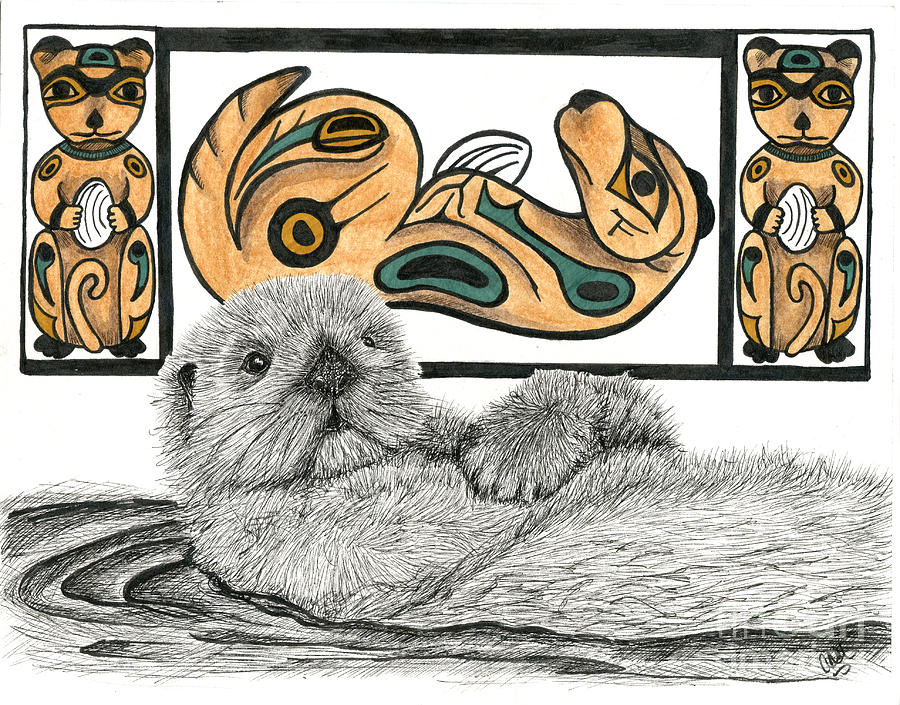This hand-drawn image features a detailed pencil sketch of an otter in the foreground, depicted in black and white, floating on his back in water with his paw resting on his belly and his head lifted. Above and behind the otter is a triptych of stylized illustrations resembling Inuit or Aztec art, featuring three brown otters accented with teal, mustard yellow, and green highlights. The left and right panels show the otters standing upright, facing the viewer, with their tails between their legs and black masks around their eyes. They hold white clamshells in their front paws and have distinctive black bands around their paws, with black-tipped ears and gold rings around their eyes. The central panel displays an otter reclining on its back, head and tail curled inward, also holding a clamshell. Each otter in the triptych has green and black nubs between their ears and intricate, elongated markings on their legs and feet. The overall composition merges the serene foreground with the vibrant, culturally inspired background, linking traditional pencil sketching with colorful, symbolic illustration.